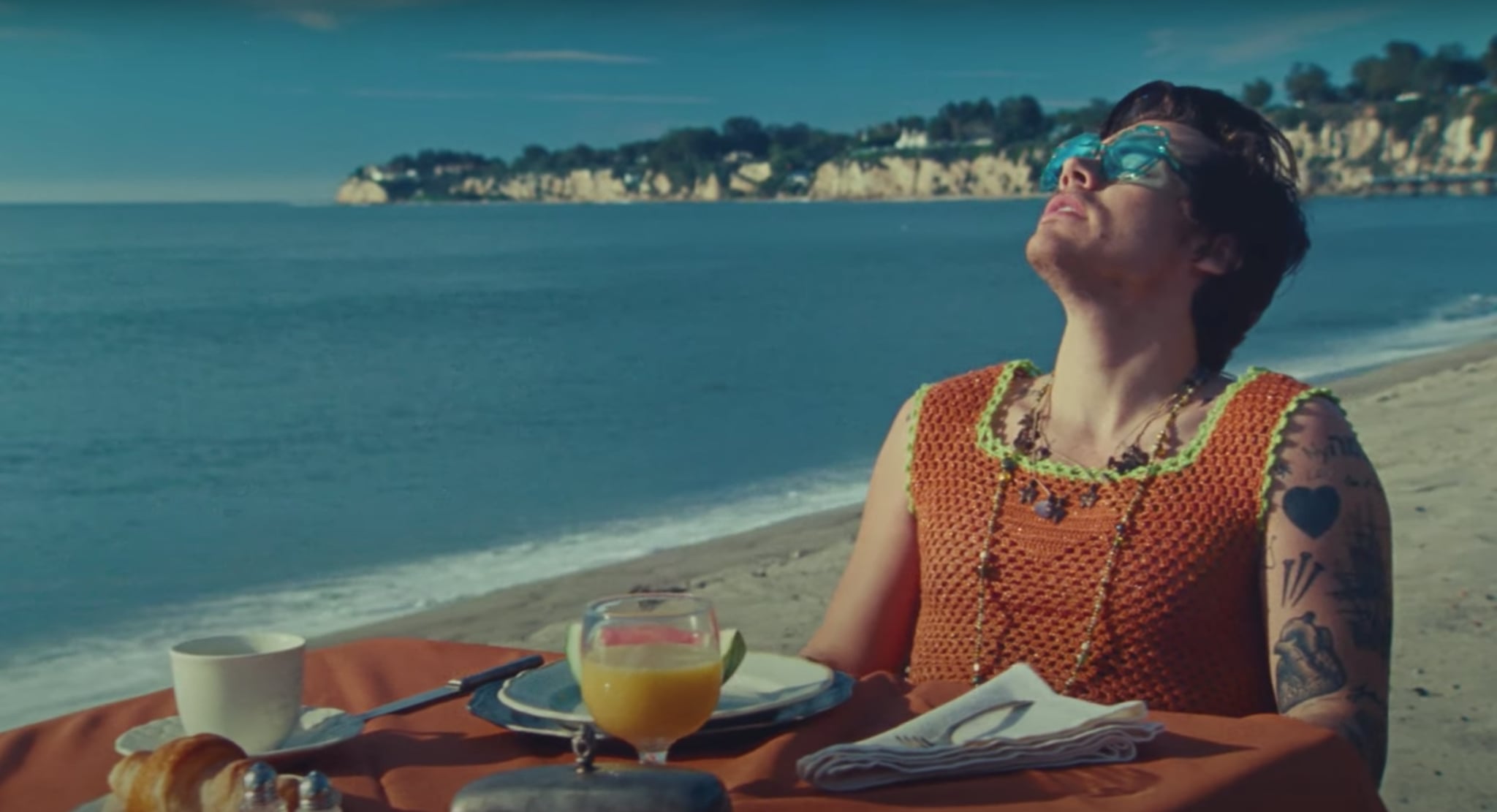In this captivating image, Harry Styles is seated at a beachside table with a beautiful blue sky meeting the serene ocean in the backdrop. His head is tilted up with his eyes closed, basking in the relaxing atmosphere. He sports stylish blue sunglasses and a distinctive orange knit shirt adorned with yellow and green borders. Around his neck, he wears two layered necklaces. The table in front of him features an orange tablecloth and is set with a variety of breakfast items such as a glass of orange juice, a croissant, a small tea set, a silver butter dish, a napkin with a fork, a knife, a silver spoon, and a plate. Tattoos, including hearts, nails, and a bird, are visible on his arm. The scenic background showcases a white sand beach with waves gently lapping at the shore, cliffs adorned with trees, and houses perched on the mountainside, contributing to a luxurious and tranquil beach ambiance.